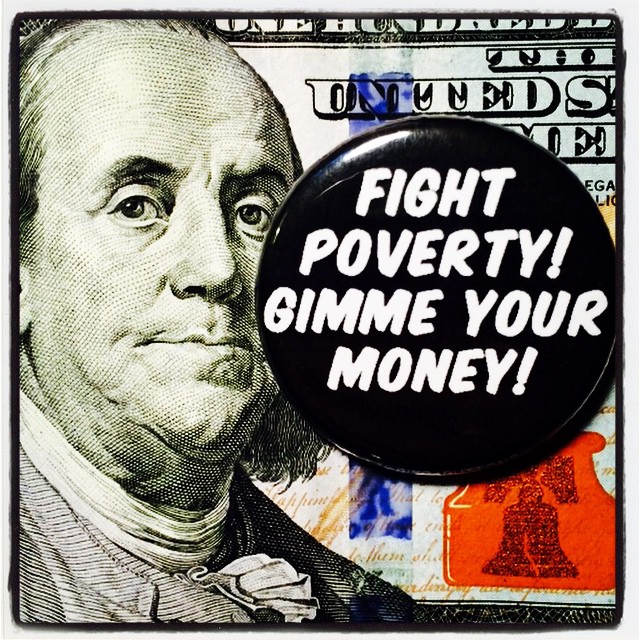This image features a close-up, edited photograph of the $100 bill, prominently displaying the portrait of Benjamin Franklin, who is looking forward wearing a white scarf and tie beneath his chin. The scene is cropped tightly, emphasizing Franklin's face while partially concealing it with a black button that humorously reads in white text, "Fight Poverty, Give Me Your Money!" The button obscures the right side of Franklin's face, particularly his right eye. Key details of the bill, such as the Pennsylvania Bell logo, orange Liberty Bell watermark, and vertical blue anti-counterfeit stripe, are visible. The upper part of the image also includes fragmentary text from the bill's top left, showing "100" and partially showing "United States."